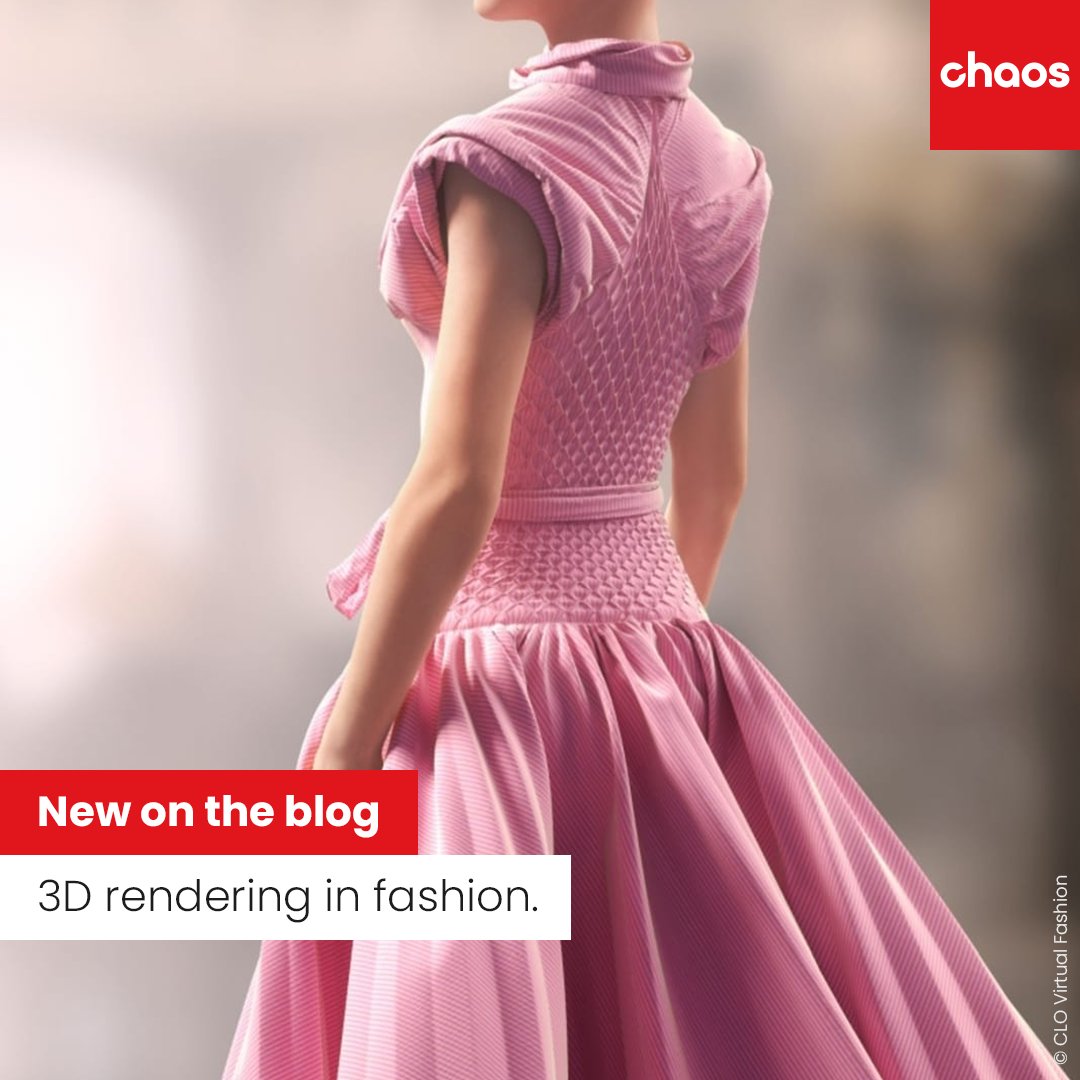The image captures a digitally-rendered advertisement, likely for a fashion blog. The focal point is a very pale-skinned female model dressed in a long, flowing, sleeveless or cap-sleeved pink dress that features a tight bodice and a pink belt at the waist. The dress extends down towards the floor with an expansive, pleated skirt. The background is fuzzy and hazy, predominantly featuring shades of pink and white, adding to the ethereal quality of the image.

In the upper right-hand corner, there is a red box with bold white letters spelling "CHAOS." On the lower left-hand corner, another red box contains the text "NEW ON THE BLOG" in white letters, and below it, in a white box with black letters, it reads "3D RENDERING IN FASHION." Additionally, the text "CLO VIRTUAL FASHION" is found along the lower right corner, suggesting that the model and dress may be computer-generated. The entire composition implies a sophisticated blend of fashion and digital artistry.